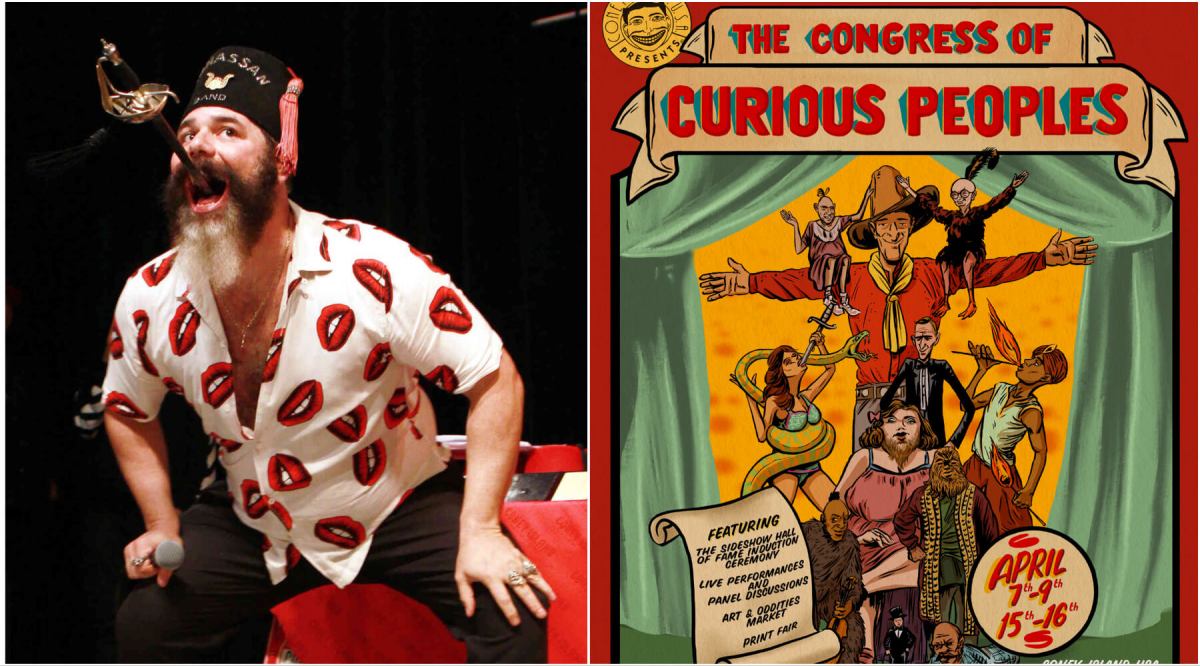The image features two side-by-side panels. The left panel is a photograph of a light-skinned man with a distinctive beard—gray in the center and black along the mustache and sides—wearing a black fez-like hat with some lettering on it. He is a performer, seemingly mid-act, with a vintage sword held in his open mouth, the golden handle visible. The man is dressed in a white, short-sleeved, button-down shirt adorned with red lips and upper teeth designs, paired with black trousers. He is in a crouched position, leaning forward, with hands resting on bent knees, and holding a microphone in his right hand.

The right panel displays a vintage-styled poster with a circus theme, titled "The Congress of Curious Peoples" in bold red letters on a beige background, divided across two yellow banners. The central figure is a cowboy wearing a red shirt, yellow scarf, and tan hat, arms outstretched, flanked by cartoon characters: a jester, a ballerina, a flame eater, and small elf-like beings perched on the cowboy's shoulders. The scene includes an Alfred E. Neuman-like face and a woman entwined with a snake. Light blue curtains frame the scene, tied back to reveal the performers. In the lower right corner, red letters denote event dates: April 7-9 and 15-16.